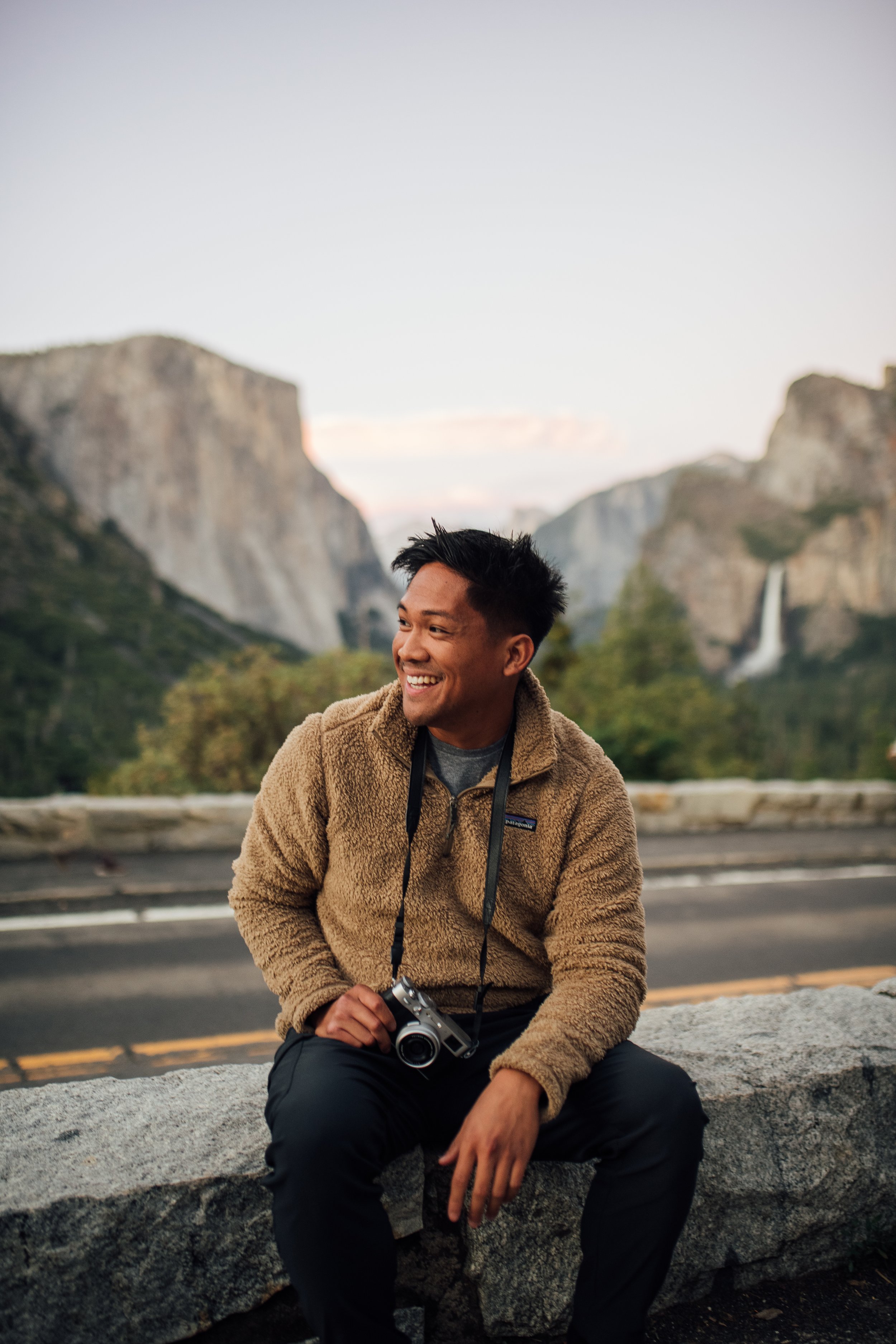In this captivating photograph, a young, light brown-skinned man is seen sitting on a stone barrier that lines the side of a road. He is smiling warmly and looking off to his left, seemingly lost in a moment of joy. The man is dressed in a long-sleeve Patagonia fuzzy sweater with a gray undershirt and black cargo pants, and he has short black hair. Draped around his neck is a modern DSLR camera with a vintage appearance, a clear indication of his interest in photography.

The scene around him is nothing short of breathtaking. Behind him, majestic rocky cliffs and mountainous landscapes, possibly reminiscent of Yellowstone National Park or Yosemite National Park, stretch into the distance. Towering stone mountains and the grassy tops of trees add an element of grandeur to the background. To the right of the man and slightly behind him is a small but enchanting waterfall, cascading gracefully and adding a touch of serene beauty to the scene. Although he does not seem to be directly admiring this stunning natural spectacle, the setting sun casts a soft, slightly dark hue across the clear sky, suggesting it is either midday or nearing sunset. The photograph captures a perfect harmony between the man's serene demeanor and the awe-inspiring natural surroundings.